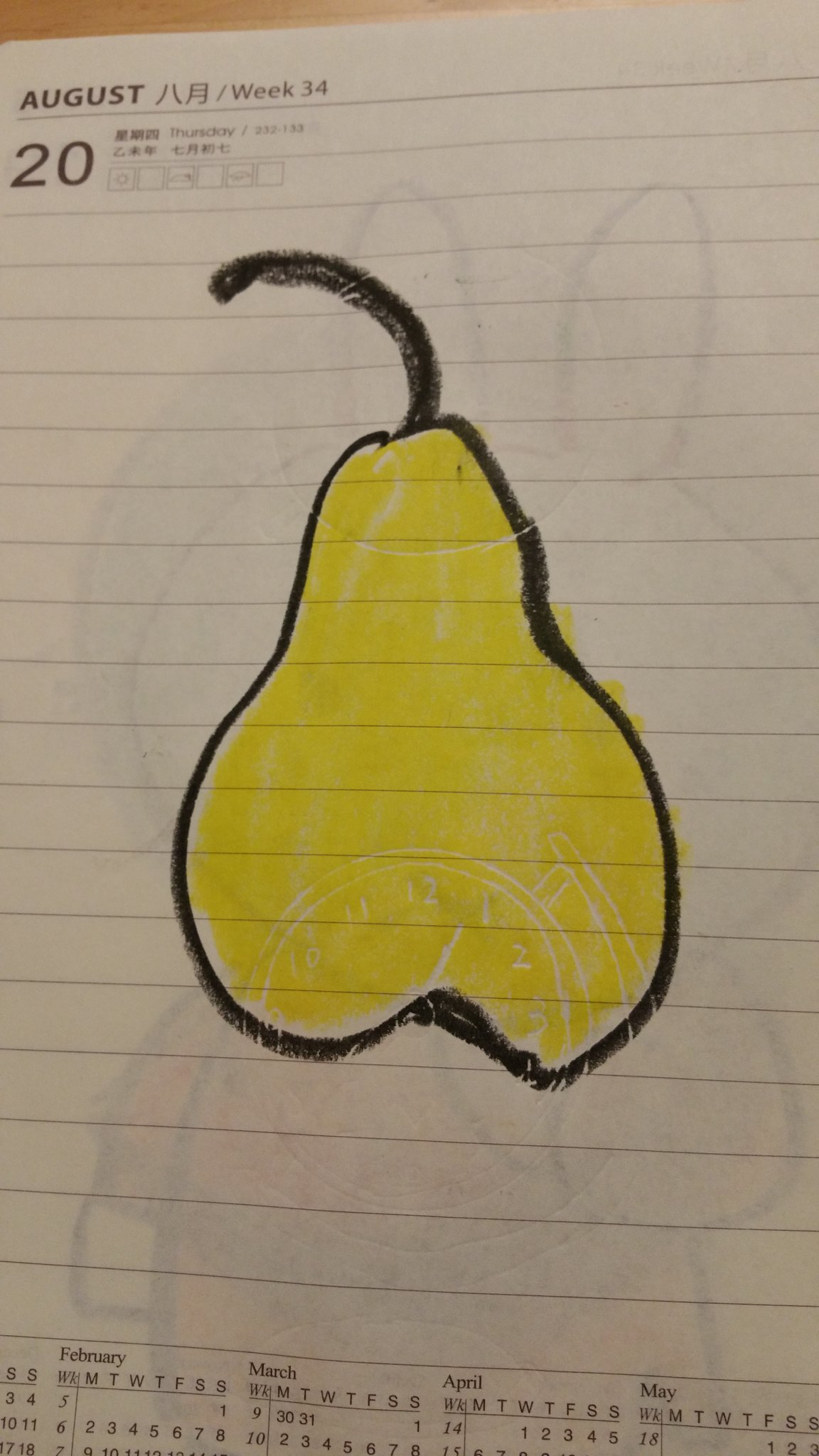This is a detailed and colorful photograph of a page from a paper desk calendar. At the top left of the page, the month "August" is prominently displayed, followed by some oriental characters, and the designation "Week 34." Just below this, the number "20" is visible along with more oriental characters, and the day "Thursday." The page itself is lined and features a bold drawing of a pear at its center. The pear is outlined in black crayon with a stem that curves to the left. The interior of the pear is roughly colored yellow, with the coloring sometimes extending beyond the black outline. Superimposed on the bottom half of the pear drawing is the top half of a clock face, revealing the numbers 10 to 3. Additionally, there is a faint bleed-through of another drawing from the reverse side of the page, hinting at a rabbit. At the very bottom of the calendar page, partial sections of the months February, March, April, and May are visible but cut off so that the entire months aren't completely shown. This image reveals a snapshot of time and creativity on a tall, narrow calendar page.